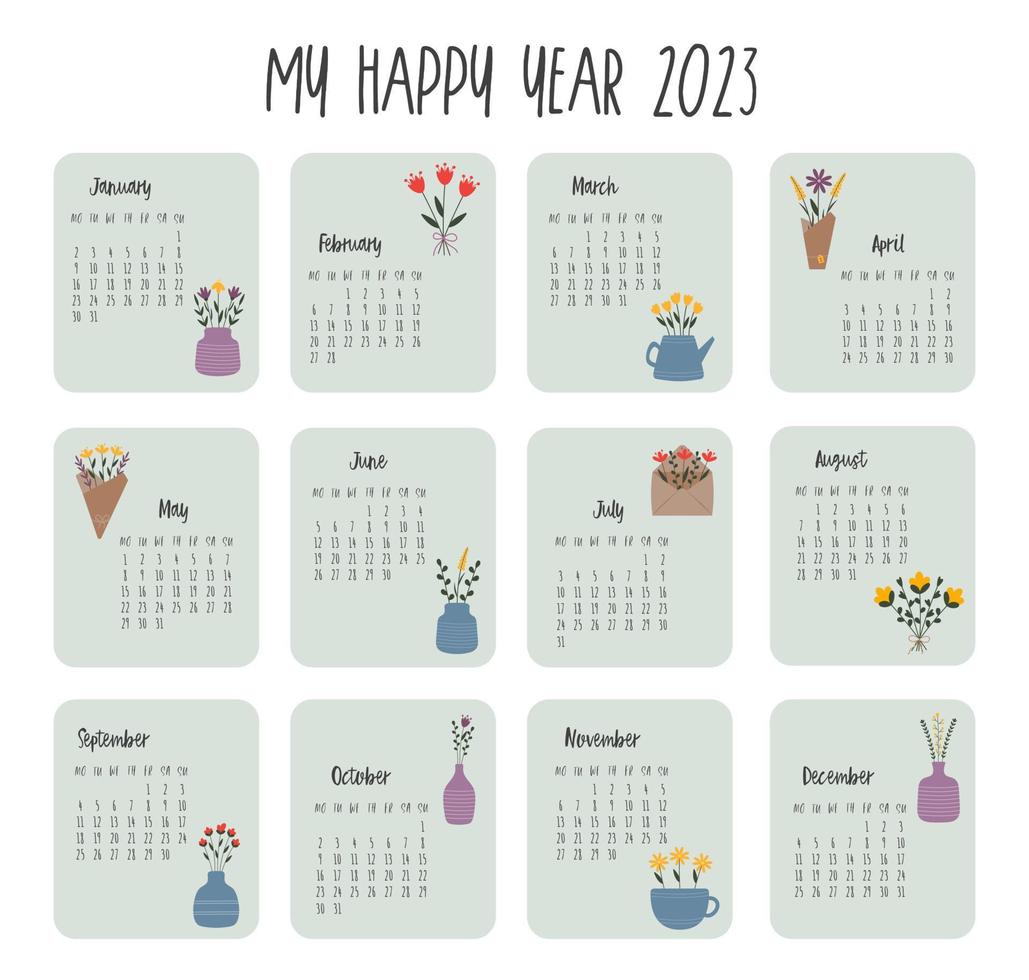The image is a meticulously designed, minimalistic digital calendar titled "My Happy Year 2023" in a thin, handwritten black font. The calendar is laid out on a white background and contains a grid of twelve squares arranged in three rows of four. Each square represents a month and features a light green background with rounded corners.

Within each month's square, the names and dates are displayed in a black, cursive, and elegant handwritten style. Each square also includes a unique botanical illustration, adding a touch of creativity and charm. For instance, January showcases a purple pot with a purple and yellow flower, located in the bottom right corner, while February features three red flowers in the top right corner.

The overall design of this calendar combines simplicity with a touch of whimsical elegance, making it both functional and visually appealing.